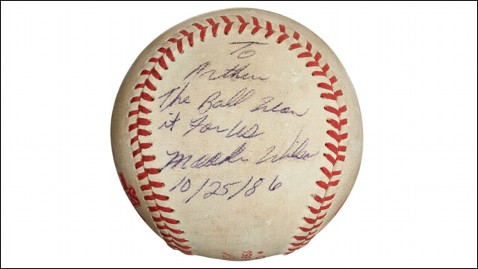The photograph showcases a standard, used baseball, displayed against a pure white background edged with a thin black line. The baseball, slightly off-white with blemishes and traces of brown from dirt and clay, bears the signature red stitching that forms an upside-down horseshoe pattern. On the face of the baseball, an autograph written in pen is partly legible: "To Arthur, the ball [unintelligible] it for [unintelligible]." The name of the signer is difficult to discern but seems to begin with "M" and include a "W." Below the inscription, the date "10/25/86" is clearly written.